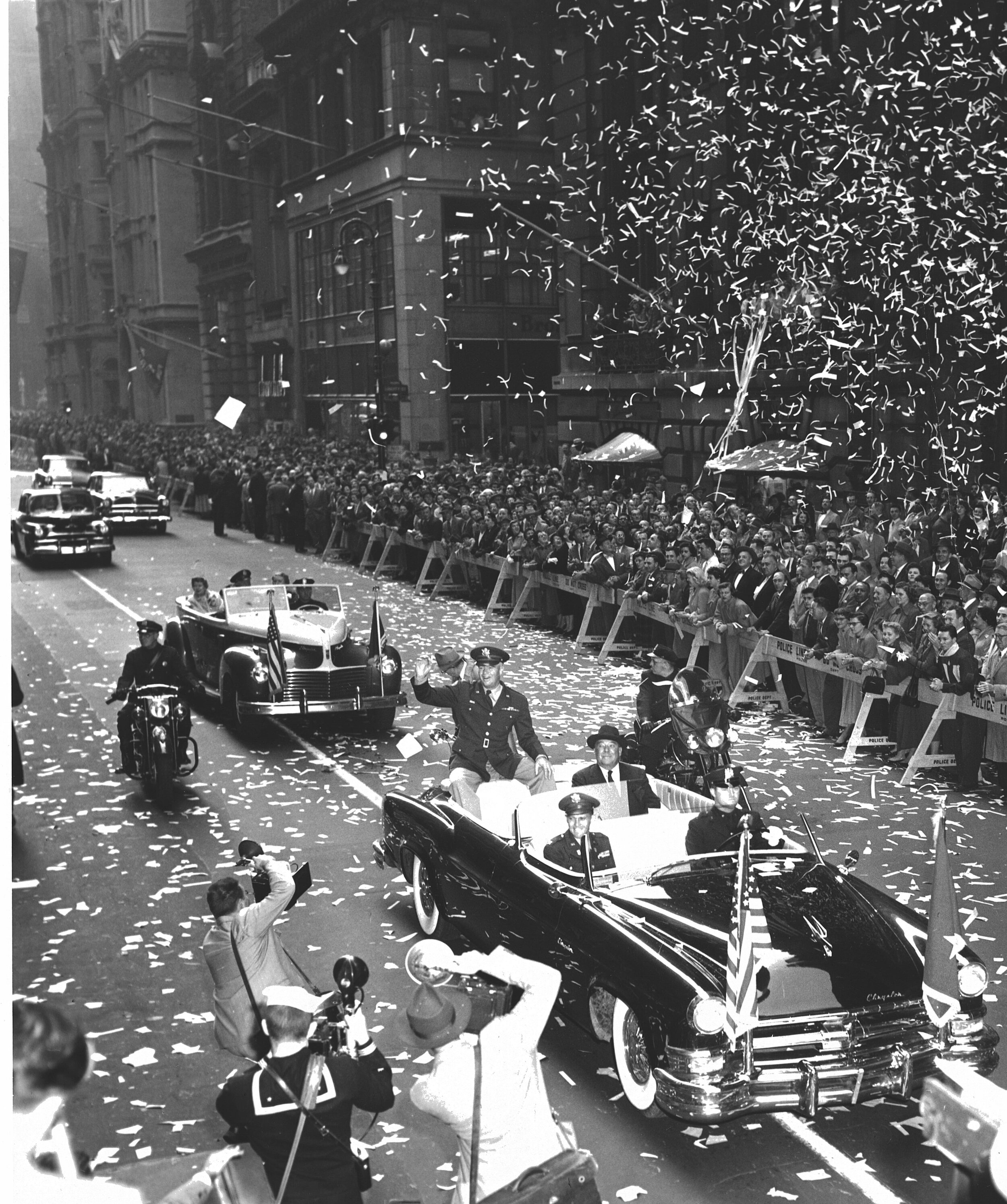This black-and-white photograph captures a lively parade, likely from the late 1940s, possibly post-World War II, in a major city such as New York City. The main street is bustling with activity, with a line of long, vintage cars progressing towards the bottom right of the frame, while more cars can be seen further back towards the middle-left. Prominently featured is an old Chrysler convertible with flags on its bumper. Military officers, in uniform, occupy the cars, and one individual is notably sitting on the top of the back seat, waving to the enthusiastic crowd.

The parade route is lined with wooden sawhorses, keeping the large crowd at bay, while a flurry of confetti fills the air and covers the street. On the left-hand side of the image, several photographers are positioned, capturing the celebratory moments. This evocative scene, filled with servicemen, vintage cars, and jubilant spectators, encapsulates the celebratory post-war atmosphere of the mid-20th century.